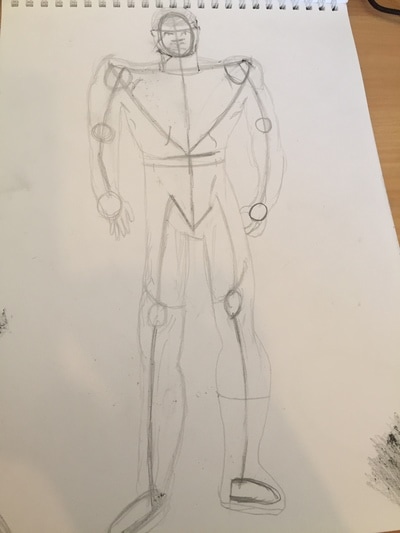The image is a detailed pencil drawing on a white sheet of notebook paper, which is held by silver coils at the top edge. The drawing occupies the entire page and features a tall, robotic man with a structured design. The figure includes a round head with a gray shaded helmet, broad shoulders, a thick neck, and a narrowed waist. The torso displays an upside-down triangle stretching from shoulder to shoulder, tapering to a point at the waist. The arms hang down by his sides, while the long legs extend to the feet, marked by ovals. The sketch's construction is mapped out with geometric shapes: circles at the joints (shoulders, elbows, knees), lines for limbs, and additional detailing layered around these shapes. The upper right corner of the page shows a triangular patch of brown, and the bottom right is shaded black. Visible through the spiral holes are small, square perforations indicative of the notebook style. The right upper corner also shows a mysterious black line, potentially a cord or hair tie.